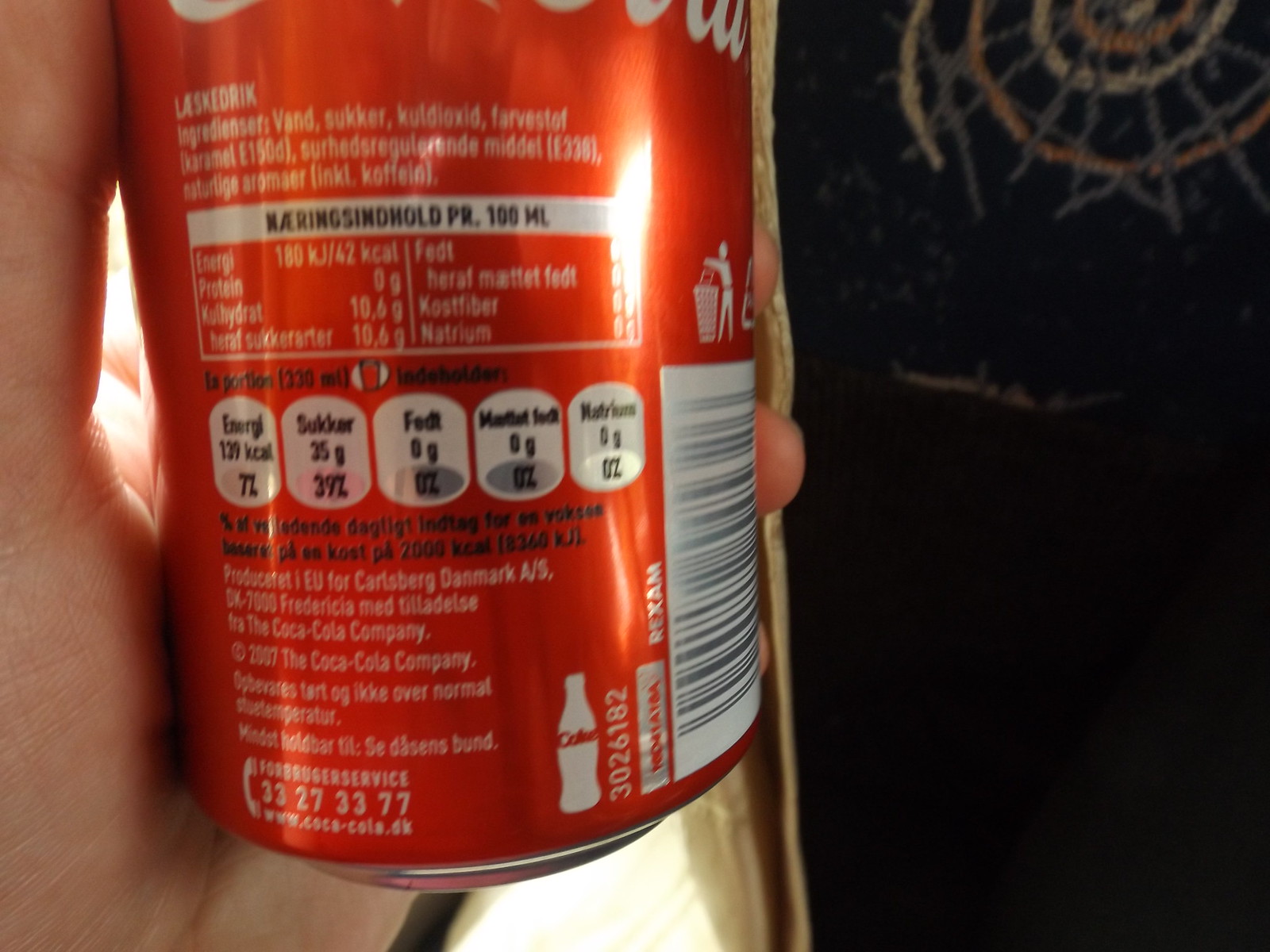In this photograph, a person is holding up a traditional red aluminum Coca-Cola can in their left hand. The can is displayed with the ingredients and barcode side clearly visible. The text on the can is printed in a language that is not understood by the viewer. The design includes the iconic white Coca-Cola script logo with red letters. Additional symbols on the can include a trash can icon, indicating proper disposal, and rounded square bubbles marking nutritional information, including grams of various contents.